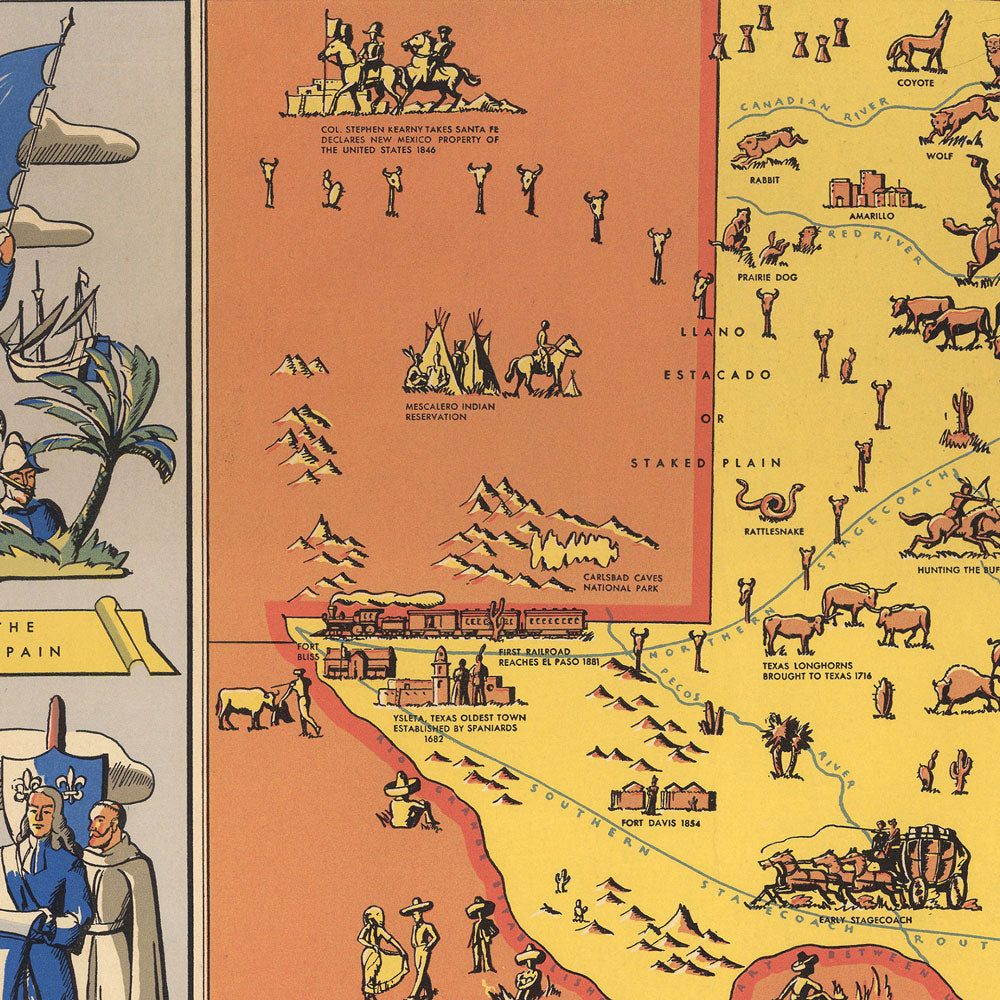This detailed illustration map combines historical and natural elements primarily of Texas, with hints of the surrounding New Mexico area. Dominating the right side of the image, Texas is marked in yellow and features a wide array of drawings and annotations, including notable landmarks such as the Carlsbad Caverns and a diverse fauna of rattlesnakes, armadillos, Texas Longhorns (brought to Texas in 1716), rabbits, coyotes, wolves, and prairie dogs. Illustrated towns like Amarillo and annotations about the Southern Stagecoach Route enhance its historic storytelling. To the left, there's an orange-hued depiction likely representing New Mexico. This section includes labels such as Colonel Stephen Kearney’s capture of Santa Fe in 1846, the Mescalero Indian Reservation with teepees and horses, and mountain ranges. Additional elements like a stagecoach, rivers including the Canadian and Red Rivers, and significant routes like the Northern Stagecoach and the First Railroad reaching El Paso in 1881, enrich the visual narrative. The upper part of this image, presented as two book pages, seamlessly blends text and imagery, adding a layer of historical context to this picturesque map.